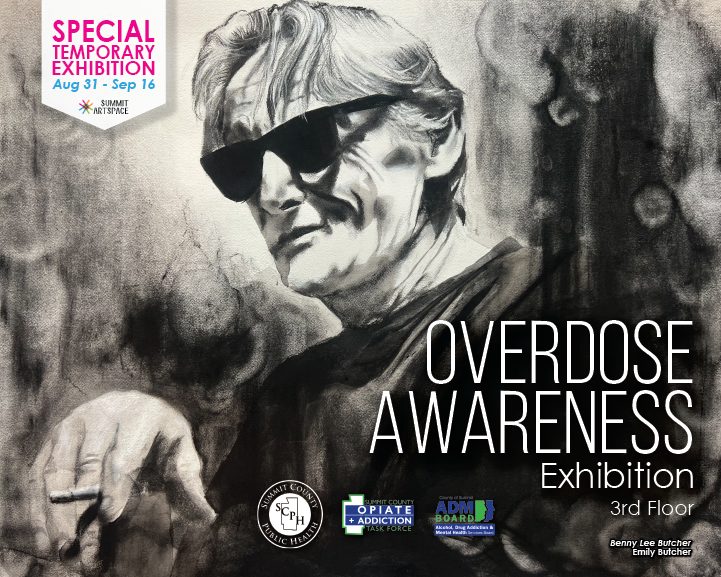The detailed image is a square, borderless poster featuring a black and white, charcoal-like illustration of a Caucasian man with shaggy blonde hair, wearing sunglasses and a black t-shirt. He is holding a cigarette between the fingers of his right hand. In the upper left corner, there is a white shield-shaped area containing text in pink and blue that reads: "Special Temporary Exhibition, August 31st to September 16th, Summit Art Space." The lower right corner of the image includes the text: "Overdose Awareness Exhibition, Third Floor," alongside the names "Benny Lee Butcher" and "Emily Butcher." Towards the bottom center of the poster, there are three logos: the first for the Summit County Public Health displayed in a circular design, the second for the Opiate Addiction Task Force, and the third for the ADM Board.